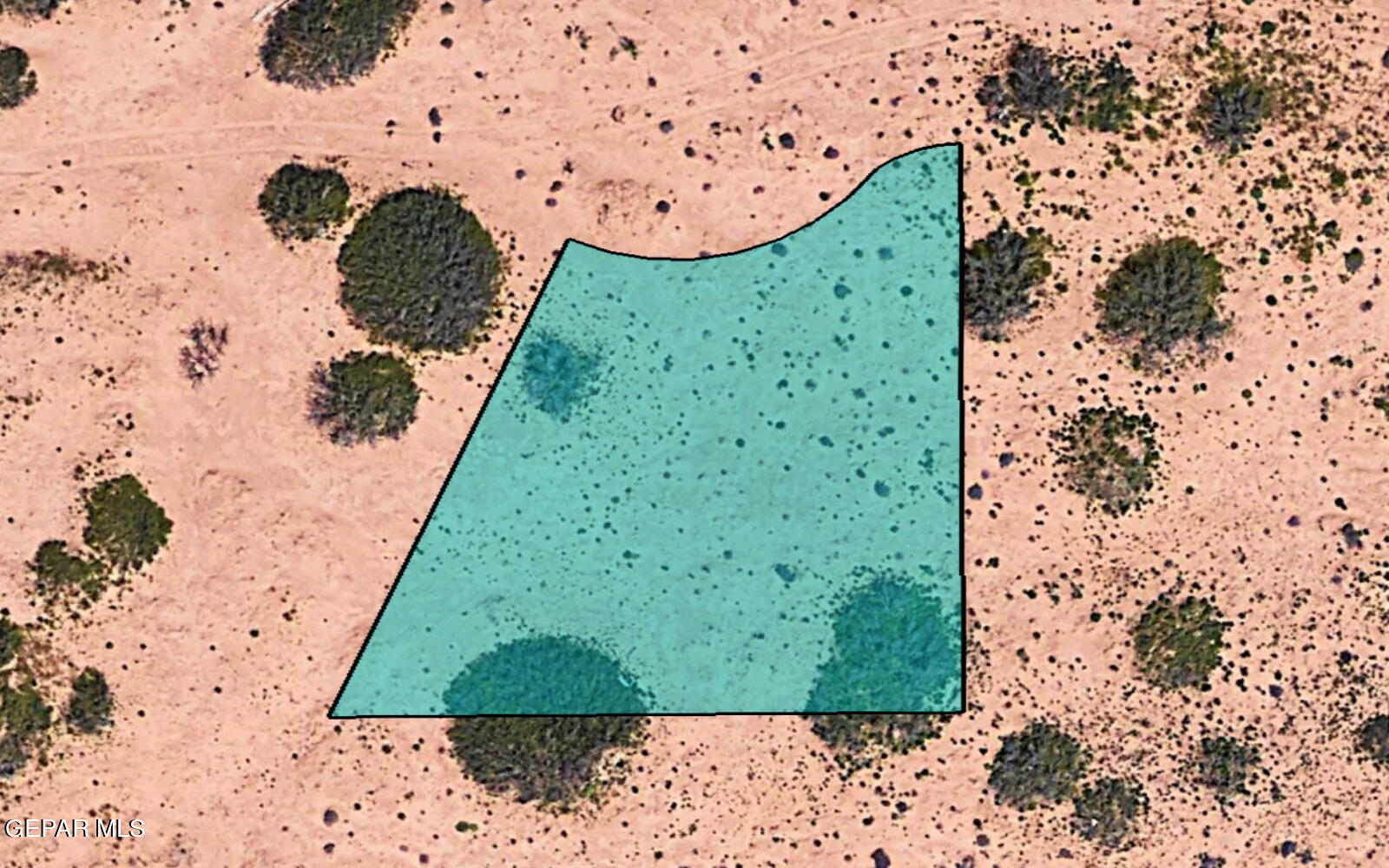This image is an overhead drone photograph of a barren desert plot of land. The ground is a light, reddish-brown color, dotted with small clumps of greenish-blue shrubbery, possibly juniper brushes, or mossy rocks scattered in circular formations. Superimposed on this scene is a transparent, teal-blue, parallelogram-shaped outline with a black border, indicating the boundaries of a specific area of land available for purchase. This outlined shape occupies about a quarter of the image, extending from an inch down from the top, stretching out to the left, forming a 90-degree angle, and then sloping down slightly as it moves toward the right. The photograph is rectangular and measures approximately six inches wide by three to four inches high. In the lower left-hand corner, the text "GEPARMLS" is displayed in white print.